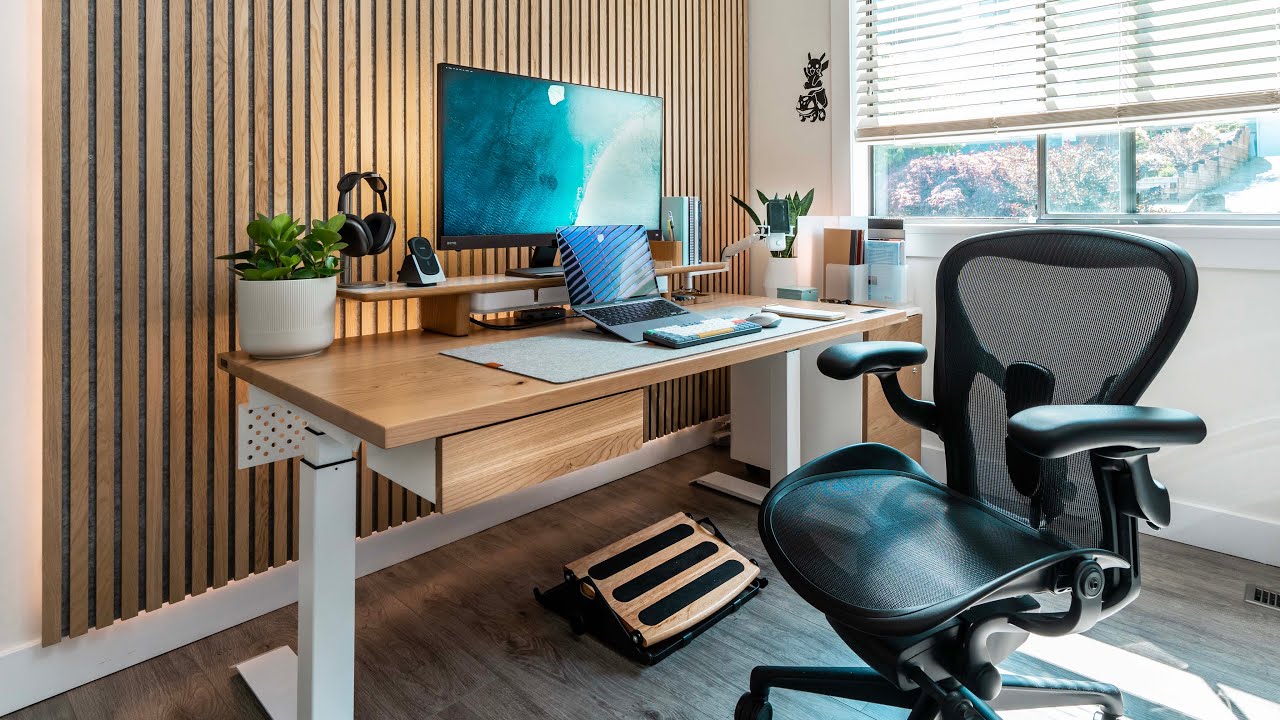The picture captures a modern, well-appointed office space. Against a background featuring a wall covered with vertical brown wooden slats framed by white borders, there is a large window with partially open blinds, allowing a glimpse of trees outside. The floor is made of brown hardwood, providing a warm foundation for the room.

In the center, a sleek, brown wooden desk stands out with its two white legs. The desk features a large, light gray, table-sized mouse pad that supports both a propped-open MacBook and a black computer monitor with a blue screen. In front of the monitor, which is notably wide, there is a mechanical wireless keyboard and an ergonomic, black mesh-back office chair that likely costs between $900 to $1,000. Underneath the desk, a brown and black footrest adds to the ergonomic setup.

On the left side of the desk sits a white pot containing a green succulent, adding a touch of nature to the workspace. Adjacent to the pot are black AirPod Max headphones resting on a wireless charging pad. The desk also has a small, brown filing cabinet with books placed on top of it.

This office setup is thoughtfully designed for both functionality and comfort, incorporating high-end, ergonomic equipment amidst a visually pleasing aesthetic.